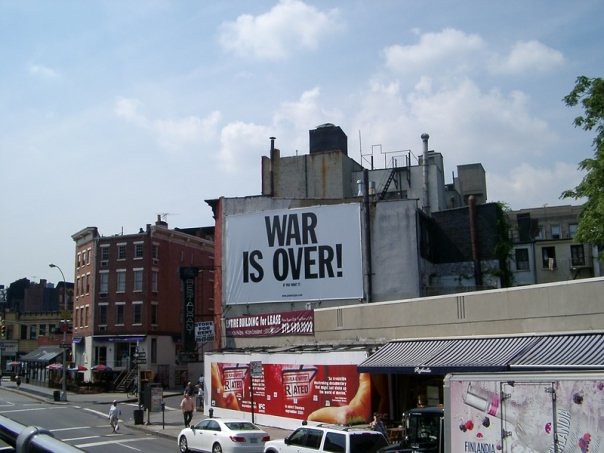The image captures a bustling street corner in what appears to be New York City. Dominating the scene is a white billboard with bold black letters proclaiming "WAR IS OVER!" accompanied by the smaller text "IF YOU WANT IT." Beneath the slogan, a partially legible website is displayed. The billboard is affixed to the side of a building characterized by a reddish brick facade and a prominent chimney. Just below the billboard, a burgundy banner announces "FOR LEASE" in white lettering, alongside additional text and a contact telephone number.

On the same building, another banner exhibits the word "RENTED" over a whitish section, potentially obscuring more information. A truck parked nearby, featuring an advertisement likely for a beverage, shares the street with a white SUV and a white sedan parked in front. The sidewalk is animated with pedestrians, including a man in a pinkish shirt and dark pants walking along the building, and another person crossing the street in khakis and a whitish shirt.

Across the way, another brick building showcases a reddish brick upper facade and a cement-like material on the ground level, decorated with window boxes filled with flowers, and a greenhouse-style area below. The street stretches further into the distance, revealing more buildings and urban elements. The sky is mostly clear with a few scattered clouds, emphasizing the pleasant weather. Notably, a tree peaks from the roof of one building, and ivy is seen climbing the rear of the building to the left, adding a touch of greenery to the urban landscape.